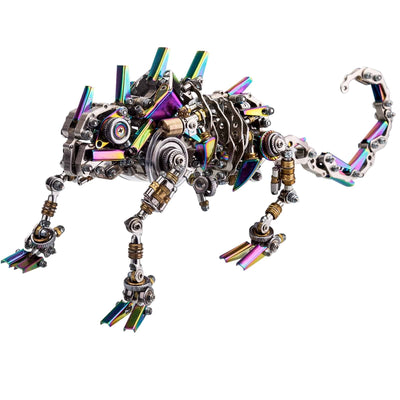The image showcases a vividly colored, robotic dinosaur toy designed for a toy or craft kit site. This mechanical-looking creature is assembled from various parts, predominantly silver, purple, and green, giving it a dynamic and futuristic appearance. The dinosaur, which resembles a lizard, stands on four legs equipped with both cylindrical gold and metallic steel components. Its feet are adorned with claws that alternate between green, pinkish-purple, and yellow hues. The creature features a long, segmented tail reminiscent of a scorpion's, adding to its unique structure. Notably, it has stegosaurus-like spiny arches along its back, primarily in green and accented with green, purple, and bluish-pink shades. The dinosaur's head houses two large, circular eyes that resemble screwdrivers, adding to its robotic aesthetic. Additionally, metallic ribs stretch across its body, contributing to its intricate and detailed design. The background is plain, emphasizing the toy's elaborate construction and vibrant colors.